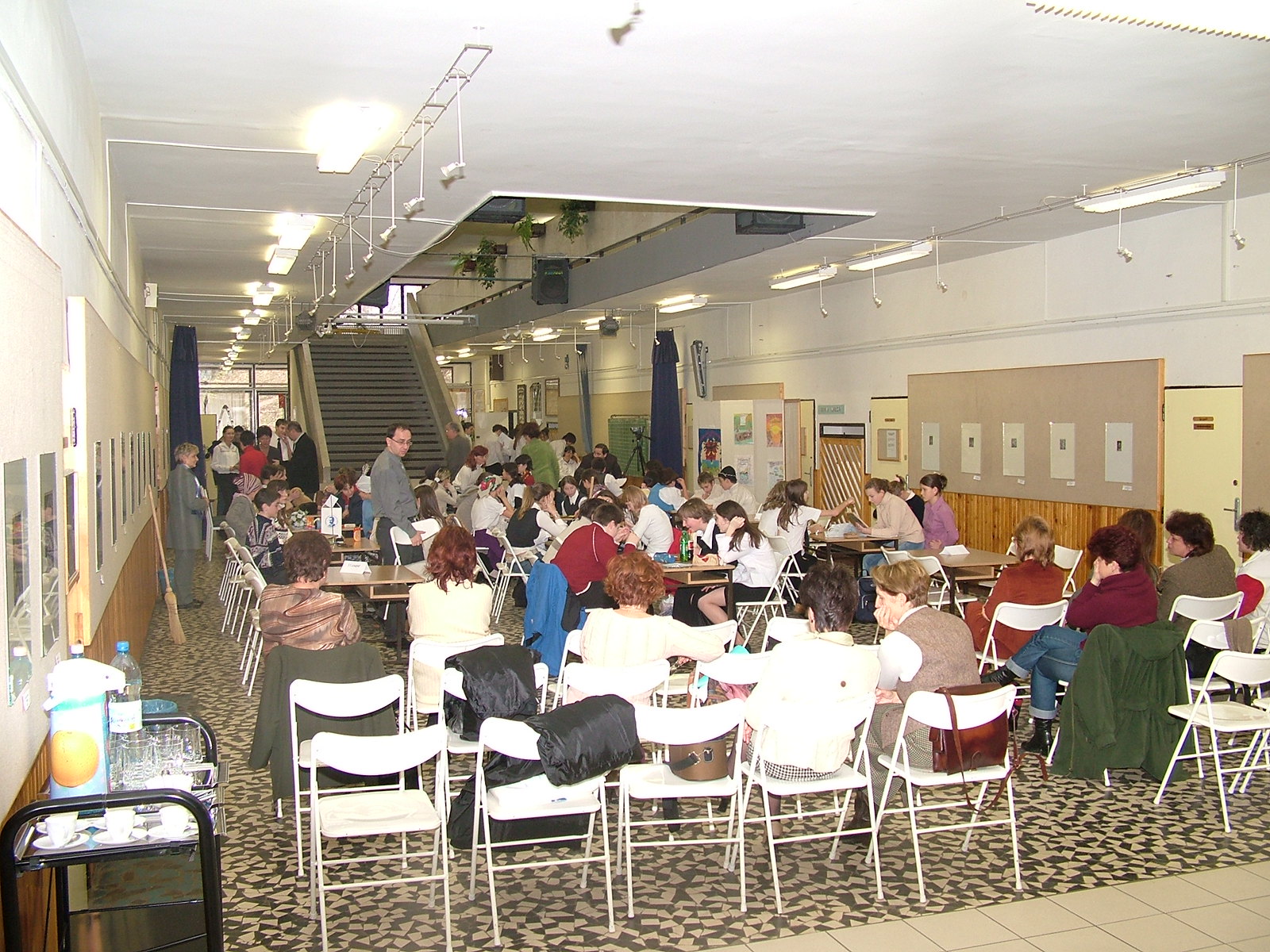The image captures a bustling indoor event set in an institutional or hospital-like space. The setting features a large room with a tiled floor partially covered by a significant carpet. Rows of white folding chairs, about half filled with spectators, are aligned facing the center where two tables are situated. Young individuals, possibly students, are gathered around these tables, seemingly engaged in an activity under the supervision of a doctor standing between them. The onlookers, who appear quite captivated, are seated along the sides and more people are seen entering from the left, gradually moving toward the tables. The background includes a staircase leading to an upper floor, with fluorescent lights illuminating the hallway which stretches out to an unseen end. Both sides of the room display identical items, such as awards or posters. The space exudes an institutional atmosphere, vibrant with varied colors like tan, gray, black, red, maroon, green, yellow, orange, purple, and blue, hinting at an engaging and diverse event.